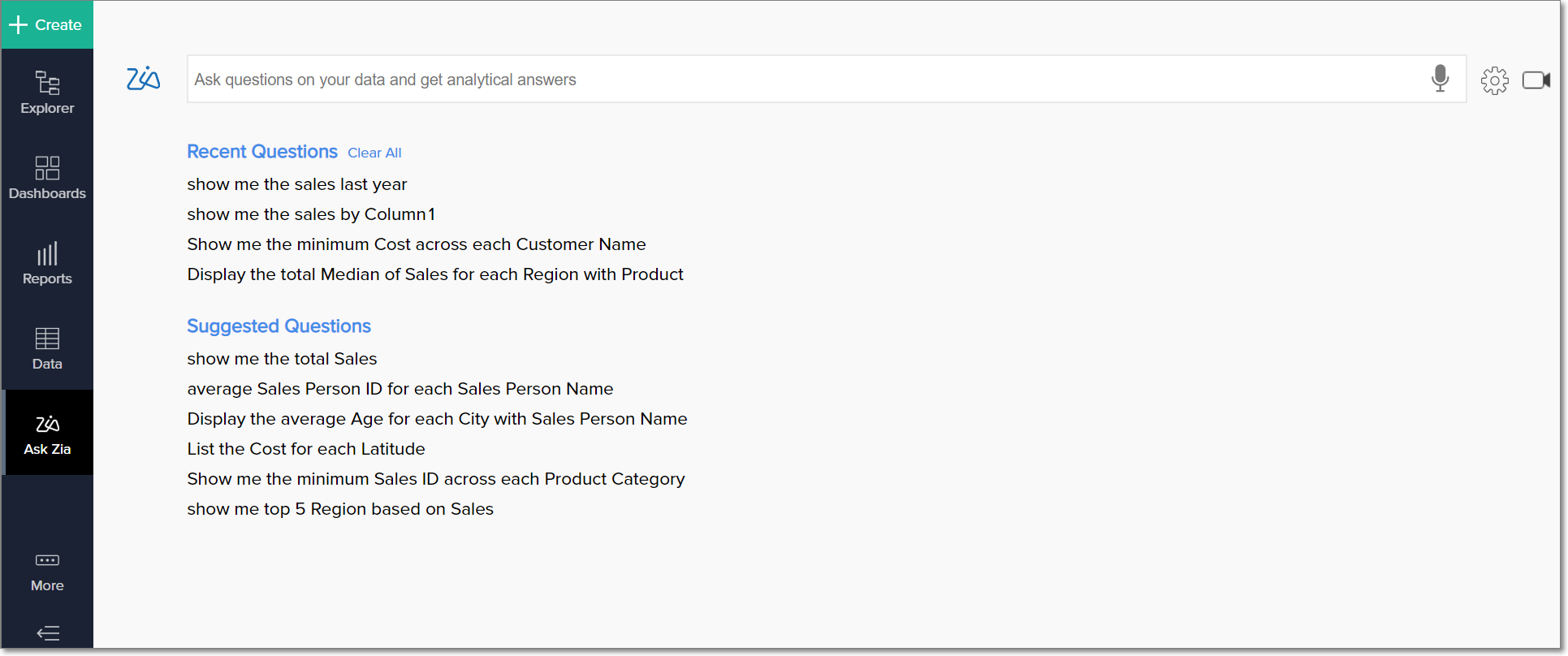A screenshot with a predominantly white background and black text is displayed. The image showcases an analytical tool’s interface, with the inscription, "Ask questions on your data and get analytical answers. Create, explore, dashboards, reports, data, ask Zia more." The tool offers sections for "Recent Questions" and "Suggested Questions," with these titles highlighted in blue for emphasis.

In the "Recent Questions" section, the user queries include:
- "Show me the sales last year."
- "Show me the sales by column one."
- "Show me the minimum cost across each customer name."
- "Display the total median of sales for each region and product."

Meanwhile, the "Suggested Questions" portion proposes:
- "Show me the total sales."
- "Provide the average salesperson ID for each salesperson name."
- "Display the average age for each city with corresponding salesperson name."
- "List the cost for each latitude."
- "Show me the minimum sales ID across each product category."
- "Show me the top five regions based on sales."

Overall, the visual is structured to help users navigate and interact with their data through intuitive, analytical queries, facilitated by the AI assistant, Zia.